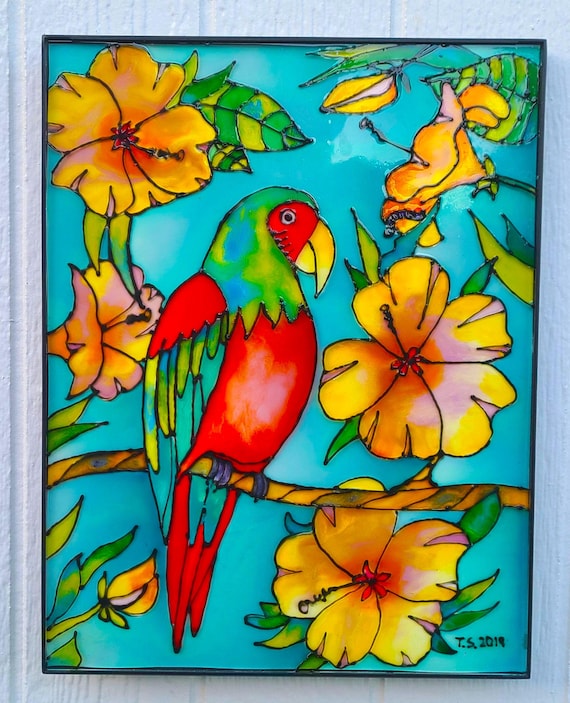Here is a detailed descriptive caption based on the given information:

A vibrant painting designed to mimic the appearance of stained glass, featuring a parrot prominently displayed in the center. The parrot, depicted in profile, showcases a rich red breast, greenish-blue neck feathers, and red face with a distinctive yellow beak. It has two black eyes bordered by white, red wings accented with turquoise, blue, and touches of yellow, and purple talons gripping a brown branch. The bird is surrounded by an array of blossoming flowers predominantly in yellow, with orange, red, and pink hues, detailed with green leaves and visible veins. These flowers form two columns flanking the parrot and extend above it, creating a natural frame. At the bottom right corner, the artist's signature "TS 2019" is inscribed in black. The artwork is framed in white with a subtle blue overtone, set against a bluish-white colored wall, giving it a glossy, stained-glass effect.